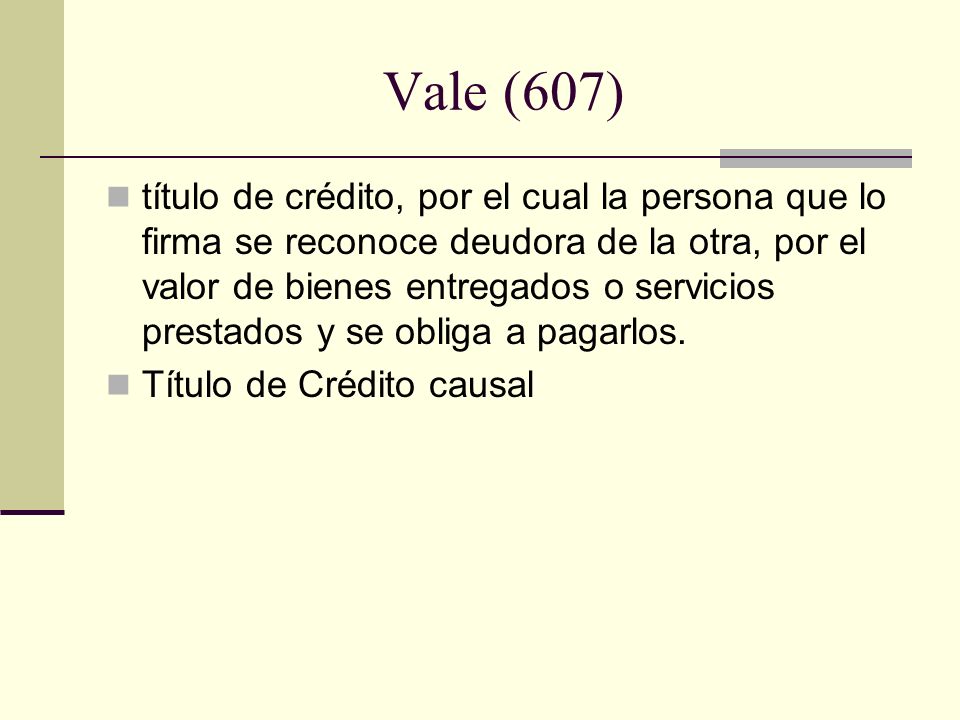The image features a pale yellow, horizontal rectangular background with a vertical column of darker yellow on the left side, occupying about two-thirds of the top portion and extending slightly past the halfway point of the image. At the top center, the title "Vale" (V-A-L-E) is prominently displayed in purple letters, followed by the number 607 enclosed in parentheses. Below this title, a horizontal purple line divides the top section from the lower portion. The lower part of the image contains two left-aligned bullet points in black font. The first bullet point states: "Titulo de credito por el cual la persona que lo firma se reconoce de dura de la otra por el valor de bienes entregados o servicios prestados y se obliga a pagarlos," spanning four lines. The second bullet point reads: "Titulo de credito casual." The text appears to be in Spanish or Italian.